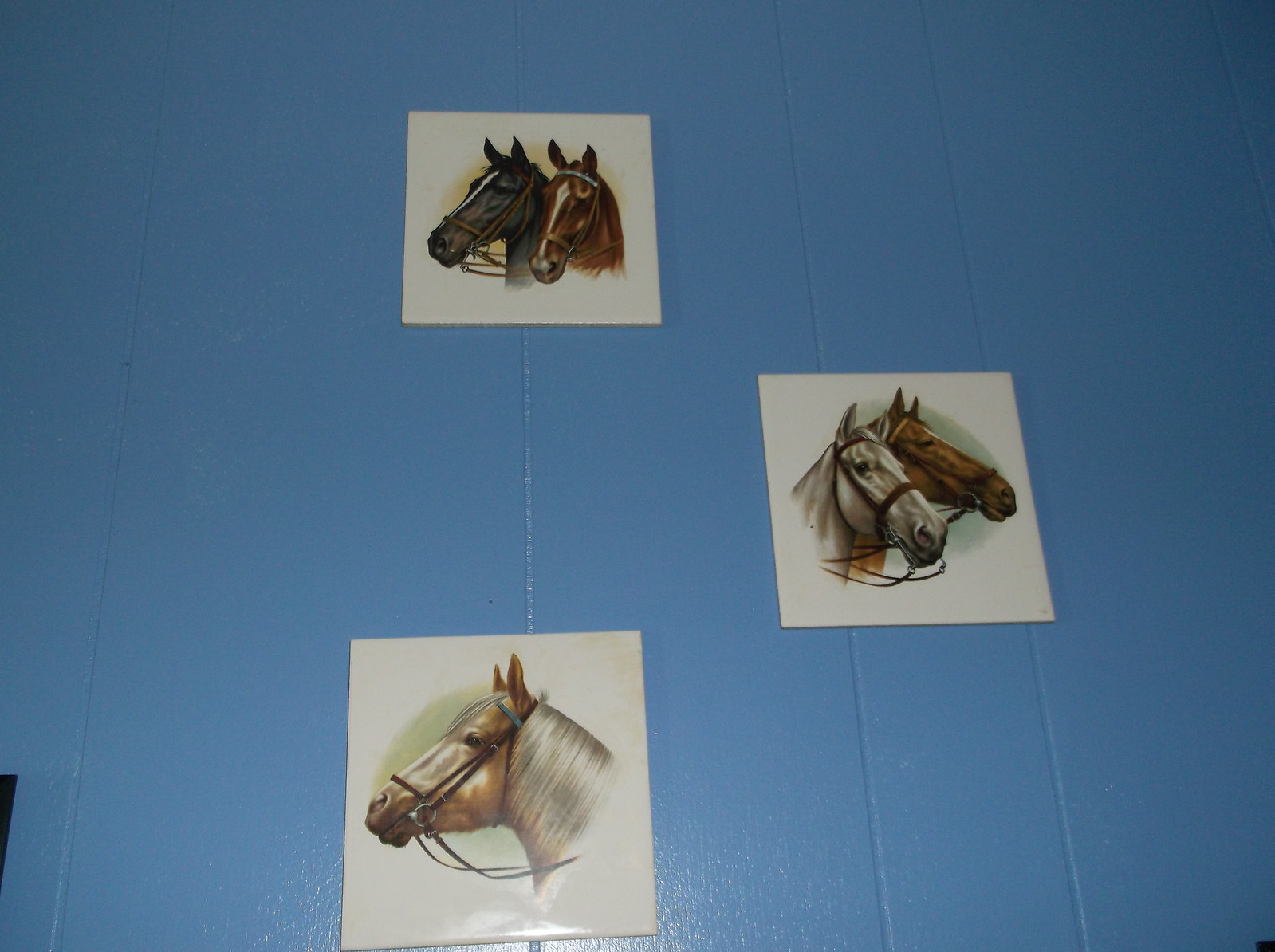This is a high-quality color photograph featuring three custom tiles mounted on a light sky blue, wooden-paneled wall. The tiles are arranged in an uneven vertical pattern: the top tile depicts two highly detailed horse heads, one brown and one black, both with white stripes down their noses, set against a yellow background. The middle tile, positioned slightly to the right, shows a white horse and a brown horse with a similar white facial stripe, both on a green background. The bottom left tile features a lone light brown horse with a flowing white mane, also wearing a harness, against a light green backdrop. All tiles are framed in white, and this image appears devoid of text, emphasizing the intricate craftsmanship and lifelike details of the horse illustrations. The photograph suggests a display of custom artwork, potentially intended for sale or personal collection.